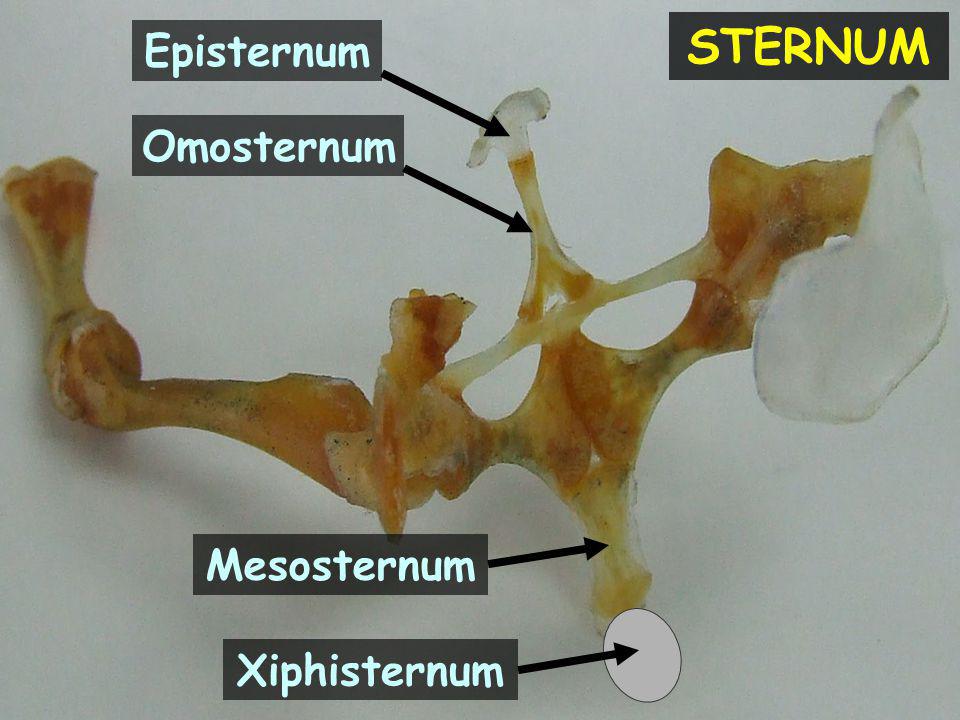The image is a detailed infographic illustrating various parts of the sternum, designed for educational purposes. In the top right corner, the word "STERNUUM" is prominently displayed in bold, yellow Comic Sans font against a black rectangular background. The main focus is a photograph of a real sternum set on a white background, with the bone appearing in shades of tan, yellowish, and dark brown. 

The sternum is divided into four labeled sections: 

1. **Episternum** - shown at the top, this part is depicted in a clear hammer shape with a black arrow pointing to it.
2. **Omasternum** - located just below the episternum, noted as the handle of the hammer, with another black arrow pointing to it.
3. **Mesosternum** - situated below the omasternum, this part has a slight yellow tint and is also marked with a black arrow.
4. **Xiphosternum** - the lowest section, indicated with a black arrow and overlaid with a white circle. 

The labels for these parts are in light blue Comic Sans font enclosed within dark gray rectangles. Only these four parts are explicitly labeled, even though the entire sternum is visible in the image. The overall presentation combines clear labeling with visual segmentation, making it an effective visual tool to understand the sternum's anatomy.